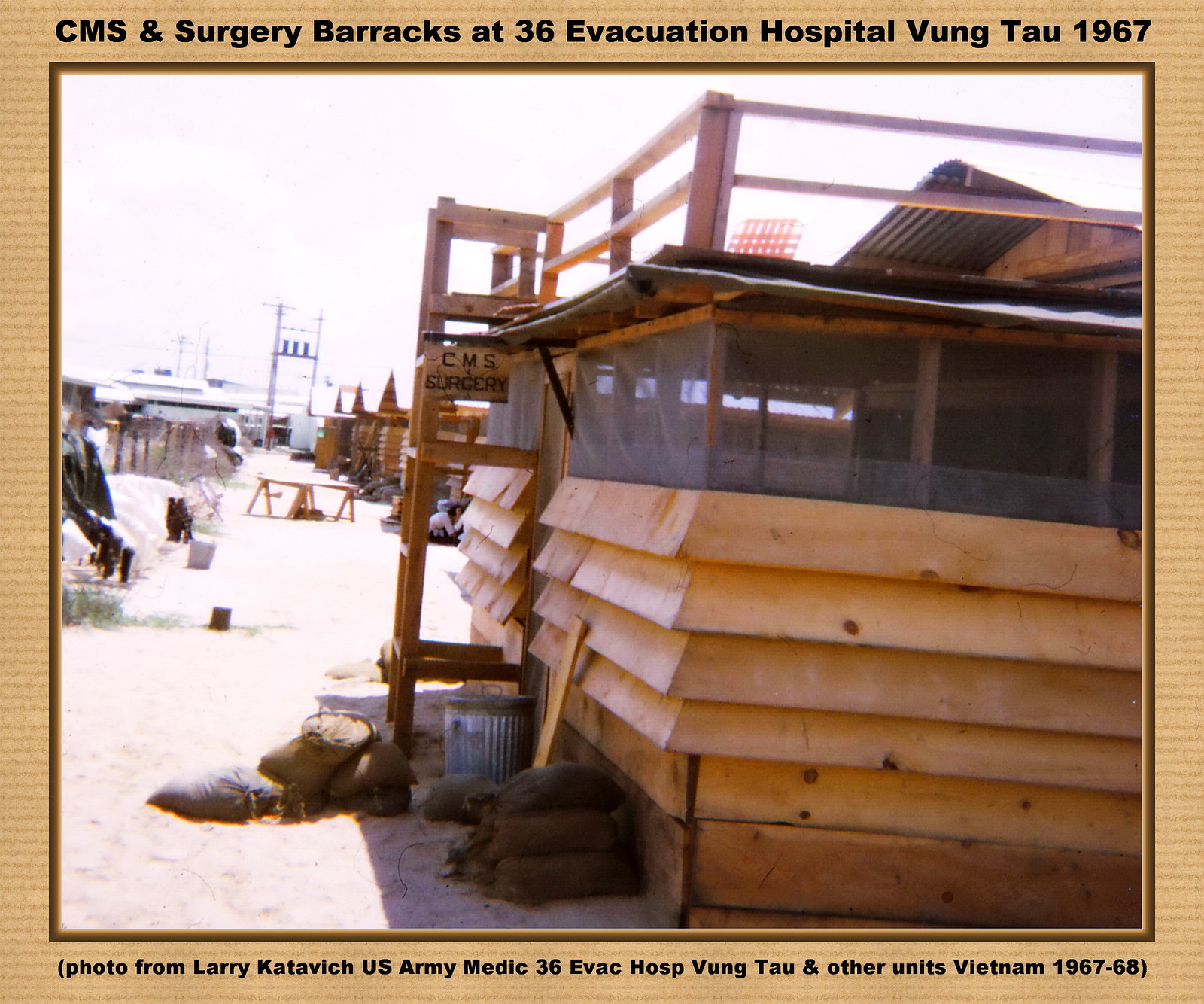The image features an old photograph from 1967, bordered by a beige-brown frame. The top of the picture reads, "CMS and Surgery Barracks at 36 Evacuation Hospital, Vung Tau, 1967," while the bottom caption states, "Photo from Larry Katovich, US Army Medic, 36 Evac Hospital, Vung Tau and other units, Vietnam 1967-68." The image itself depicts a makeshift military structure, partially constructed from wooden planks and netting, situated on sandy ground. In the foreground, there are sandbags or brown bags, a metal trash can, and scattered debris, capturing the scene's rough and utilitarian nature. The building, which has "CMS Surgery" painted on its exterior, appears weathered and surrounded by similarly shaped structures. The backdrop is brightly lit, suggesting a sunny day, casting light over the area and adding to the sense of a busy, yet stark, wartime setting.